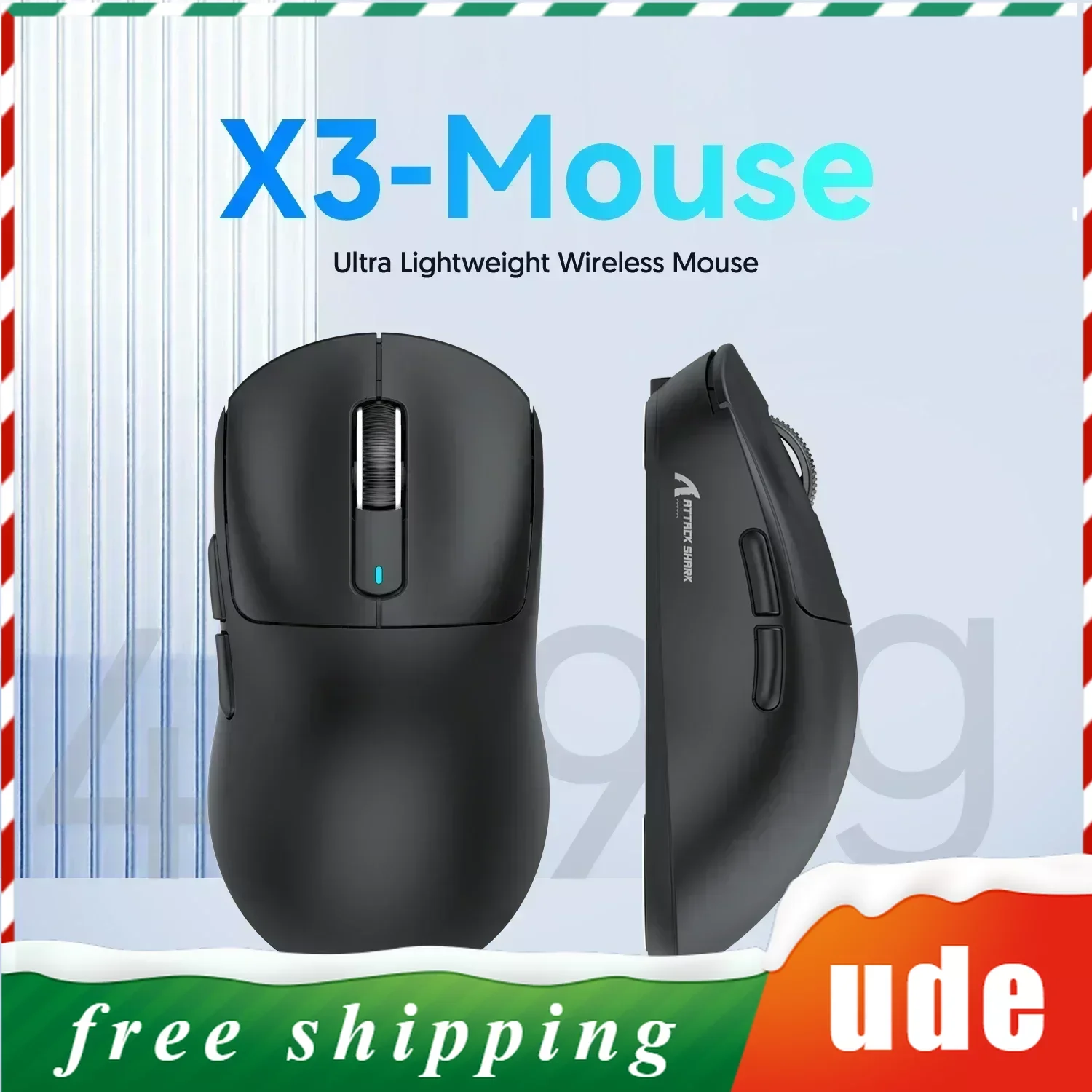The image is a high-resolution advertisement for the X3 Mouse, an ultra-lightweight wireless mouse. The title "X3 Mouse" is prominently displayed at the top in bold blue and light-blue letters, with a subtext that reads "Ultra Lightweight Wireless Mouse." The advertisement features two detailed photos of the mouse: a head-on view showing its black color, two main buttons, middle scroll wheel with a small blue LED light underneath, and two additional buttons on the side; and a side profile of the mouse. The image is framed with a festive candy-cane border consisting of green, red, and white stripes, suggesting a holiday theme. At the bottom of the ad, a green wavy banner with white text announces "free shipping." Beside it, an orange-red background displays the letters "UDE," indicating a possible company name or brand reference. There is also a light snowfall effect present above the bottom banners, enhancing the holiday feel.